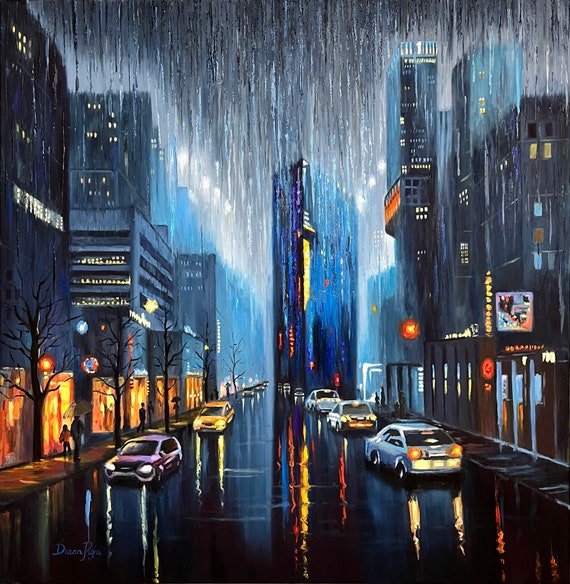This painting vividly captures a rainy night in the city, viewed from the perspective of someone standing at the end of a street. The scene is dense with reflective surfaces, emphasizing the wetness of the pavement which has a mirror-like quality. Cars traveling in both directions adorn the two-way street; on the left, three silver cars are heading away from the viewer, their red taillights glowing amidst the rain. On the right side, a red car and a yellow taxi are approaching. 

The buildings lining the street frame the urban landscape with their illuminated windows and backlit signs, giving a sense of warmth amidst the cool rain. Particularly notable is a building on the right side, possibly housing a restaurant, though the signage is difficult to read. On the left, a series of storefronts on the ground floor emit a soft orange glow through their glass and metal facades, adding to the overall ambiance of the scene.

In the background, three towering skyscrapers pierce through the rainy haze, further accentuating the city's scale and depth. The artist skillfully employs blurriness and reflective techniques to convey the incessant rainfall, with streaks of rain visible throughout the upper part of the image. People are depicted walking on the sidewalks, some carrying umbrellas, adding life and motion to the serene, wet night.